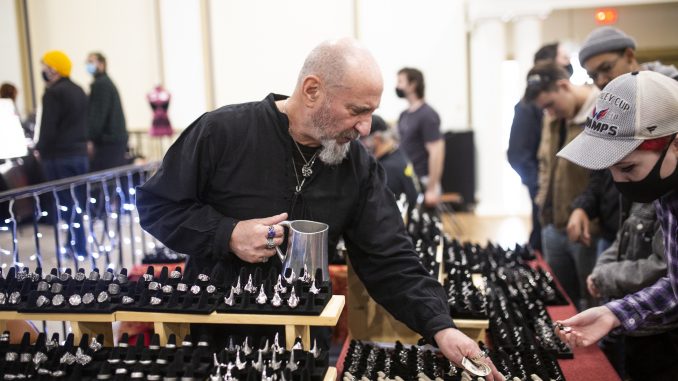In this detailed indoor scene, we see an older man with a gray beard and a bald head standing at a booth inside what appears to be a large wholesale jewelry store, bustling with people of diverse backgrounds. The gentleman is dressed in a black long-sleeved shirt and adorned with multiple rings on his fingers and a silver necklace. He holds a silver metal coffee cup in one hand and cash in the other, and seems to be engaged in selling jewelry, with various pieces displayed around him in black ring holders. Close to him, a woman is intently examining some jewelry; she is wearing a "Stanley Cup" hat, a black face mask, and a plaid flannel shirt. The background reveals an expansive room filled with other customers, some masked, perusing the jewelry displays, with an orange-globed light source illuminating the scene, highlighting the busy and vibrant atmosphere of the indoor setting.